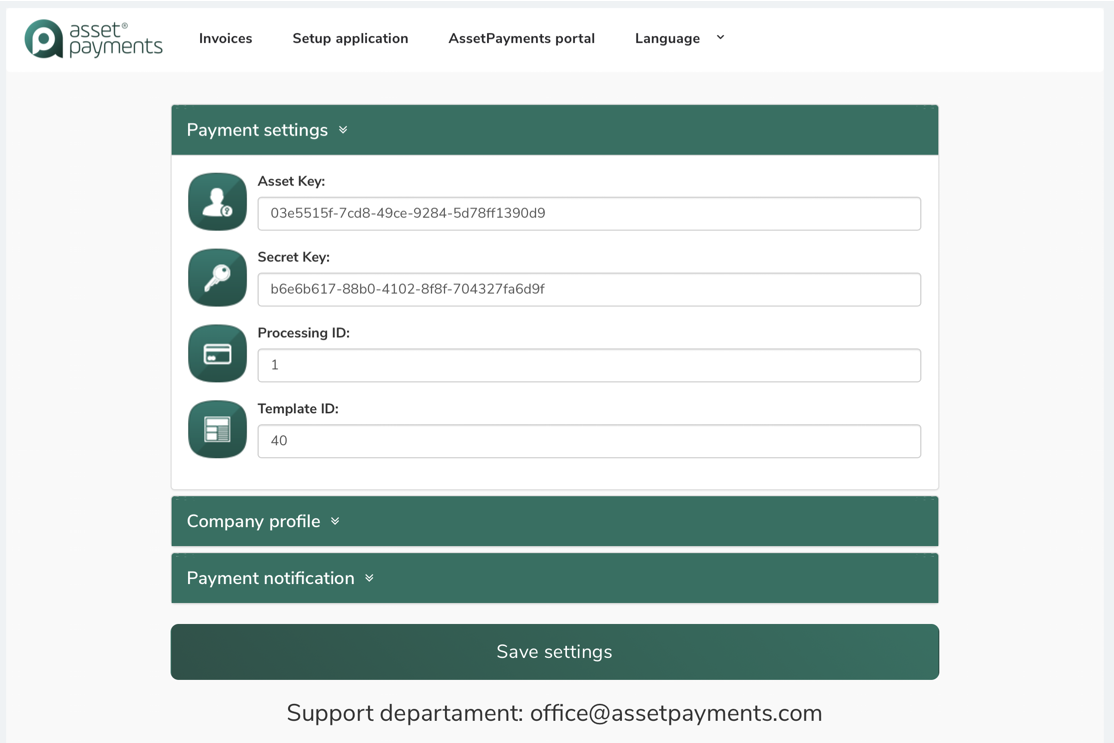Detailed Caption: 

The image displays a comprehensive interface for managing asset payments and related financial operations. On the screen, there are options to handle invoices, set up applications, and navigate through the asset payments using a dedicated portal. The interface allows the user to switch between different languages.

Key details include:
- Asset Key: 03E5515F-7CD8-49CE-9284-5D78FF1390D9
- Secret Key: B6E6B617-88BO-4102-8F8F-704327FA6D9F
- Processing ID: 1
- Template ID: 40

The company profile section features two drop-down arrows for intricate settings adjustments, similar to the payment notification section which also includes two drop-down arrows. Users can save their settings via a designated "Save Settings" button. 

For further assistance, the support department is accessible at the email address: office@assetpayments.com.